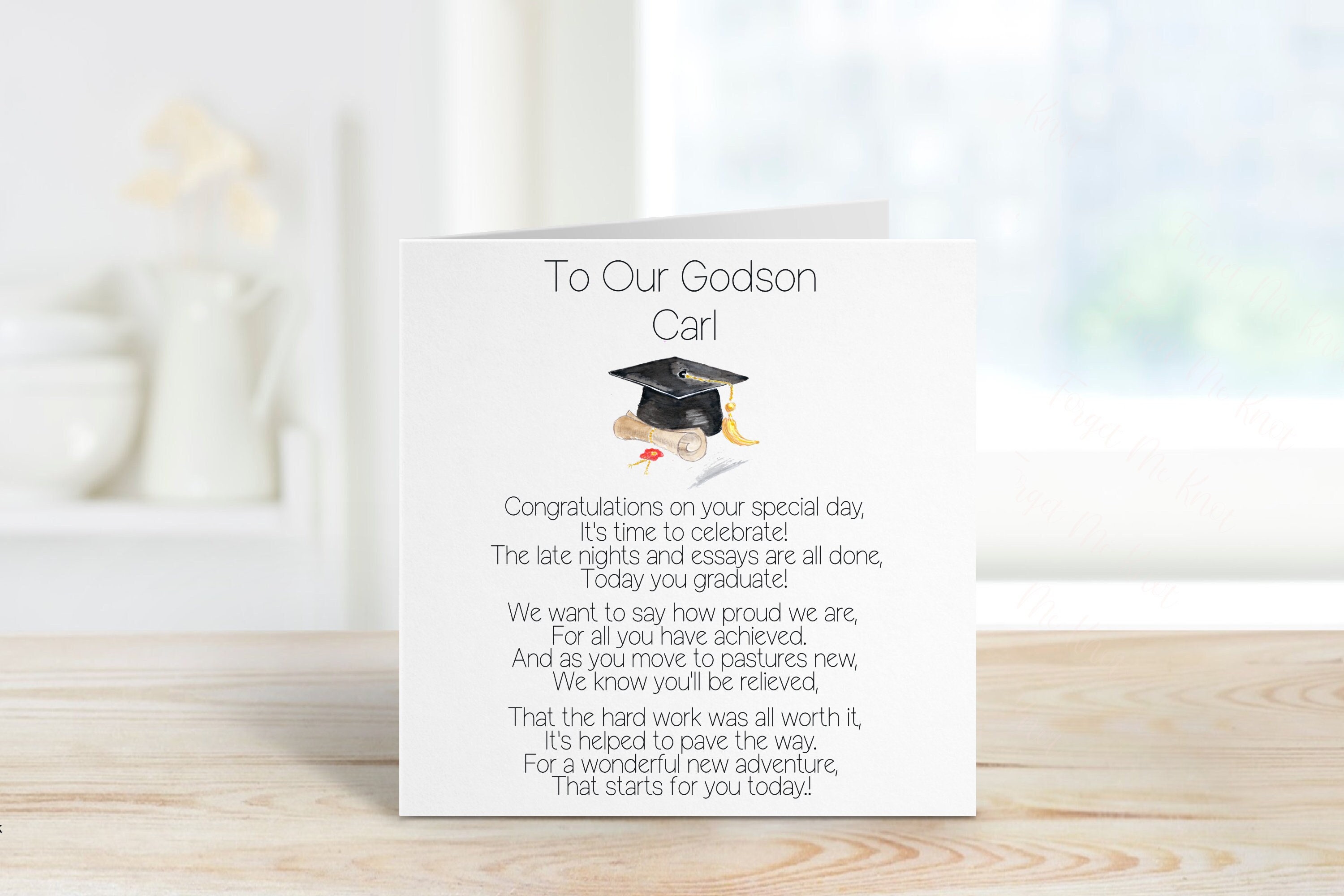A white greeting card sits slightly open on a light brown wooden table, serving as a mock-up advertisement. The card features thin black text at the top that reads, "To our grandson Carl," though other mentions imply "godson Carl." Below the text is a watercolor illustration of a graduation cap with a golden tassel on the left and a rolled-up diploma on the right. The card's message reads: "Congratulations on your special day. It's time to celebrate. The late nights and essays are all done. Today you graduate. We want to say how proud we are for all you have achieved. As you move to new pastures, we know you'll be relieved that the hard work was all worth it. It's helped to pave the way for a wonderful new adventure that starts for you today."

The background is out of focus, hinting at a domestic setting, possibly a kitchen. On the left side, there's a white wall with a white pitcher holding yellow flowers and some white bowls nearby. On the right side, a window slightly shows green leaves through its blurry glass.